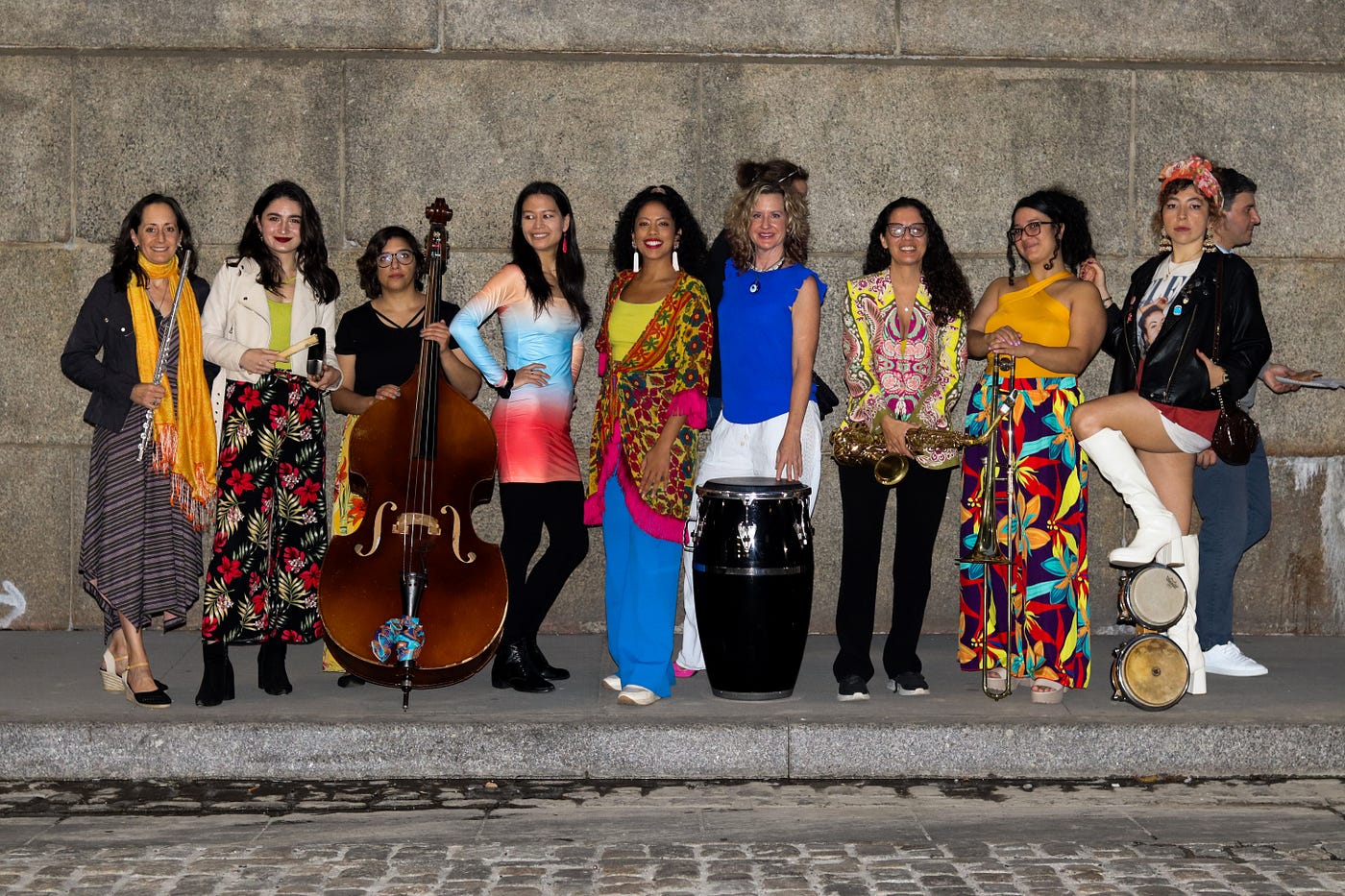In this vibrant outdoor scene, a diverse group of musicians stands proudly against a backdrop of massive grayish-tan stone blocks. The gray concrete sidewalk contrasts with the cobblestone road that lies just in front of them. Dominated by women, the ensemble also includes one man positioned subtly on the right.

Each musician brandishes her instrument with poise: the woman on the far left, distinguished by her long yellow scarf, gray jacket, and gray and black striped skirt, holds a flute. A woman next to her in a white jacket, lime green tank top, and floral black pants adds more color to the scene. The instruments they showcase include a bass, a large black drum, a saxophone, a trombone, and two small drums.

The women’s attire is as varied and vivid as their musical talents: floral dresses, blue and white pants, a black jacket paired with a red skirt, and a striking pink, orange, red, and blue dress all contribute to the colorful tableau. All are smiling and gazing directly into the camera, radiating confidence and joy. The man to the right blends into the background, adding a subtle touch to this dynamic group of musicians.